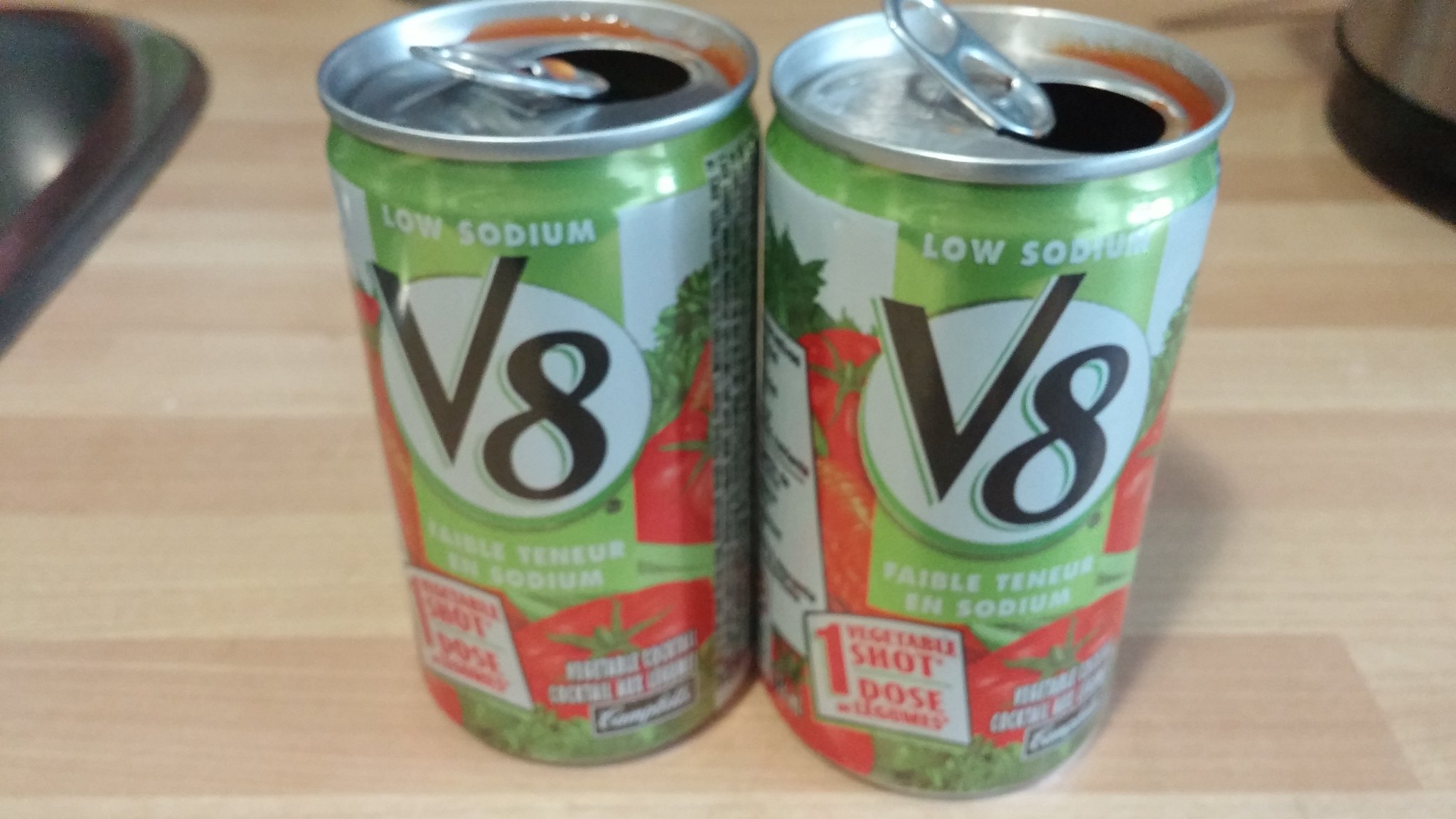This is a detailed digital photo taken indoors, focusing on two small, open V8 cans placed on a wooden countertop with a slight tan hue. The cans are light green with a white circle in the center, featuring a large black "V" extending into an "8," overlaid with the text "low sodium" at the top and images of red tomatoes around it. The aluminum cans have pop tops, with some red V8 liquid pooled around the opened rims. In the upper left of the photo, a silver-colored object resembling a stainless steel sink is visible, while the upper right features a cylindrical appliance with a black base. Additional text on the cans mentions "one vegetable shot" in a white square outlined in black.